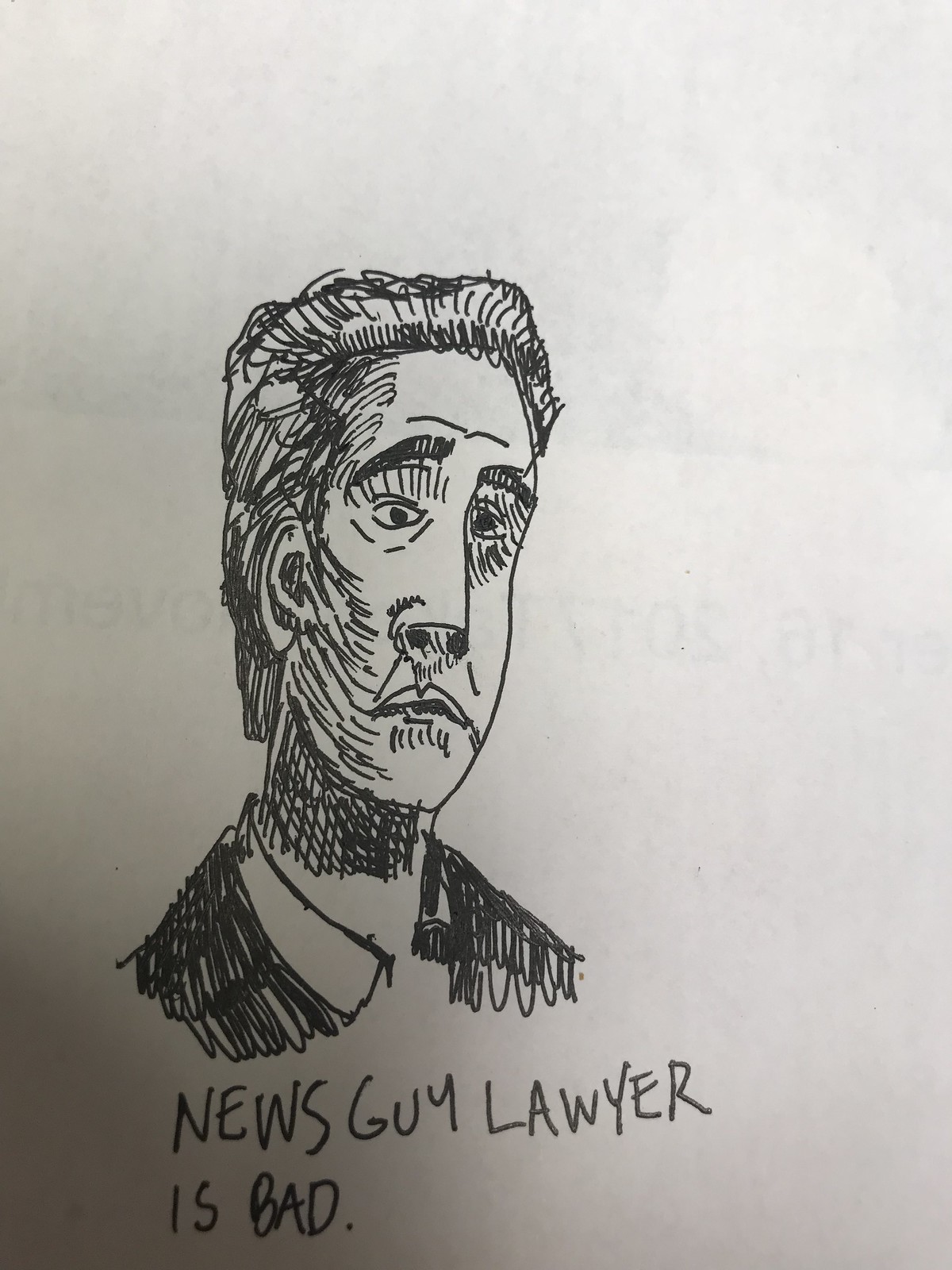The image depicts a detailed black-and-white drawing of a man, seemingly done in pencil or black ink, on light orchid-colored paper. The man, portrayed from the head down to the shoulders, is wearing a dark suit with a white collar but no visible tie or buttons. He has short, dark hair, pronounced eyebrows, big eyelashes, and lines across his forehead suggesting a state of surprise or upset. His eyes reflect a troubled expression, complementing his downturned mouth that forms a frown. The man’s long nose and thin lips also add to his displeased appearance. Below the drawing, in all capital letters, is the inscription: "NEWS GUY LAWYER IS BAD."